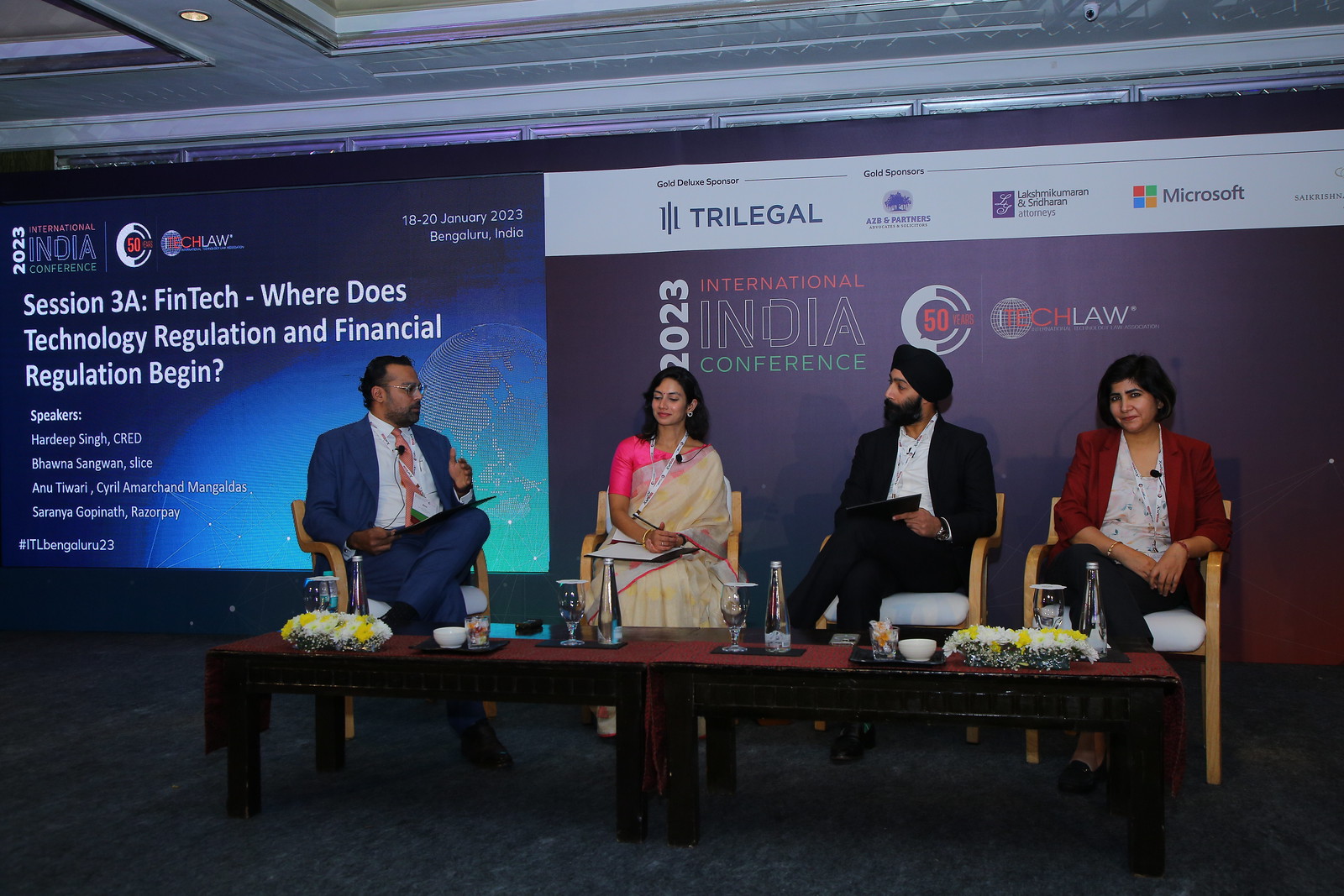This photograph captures a key moment at the 2023 International India Conference, during Session 3A on FinTech, titled “Where Technology Regulation and Financial Regulation Begin.” The event background features two large projection screens displaying crucial information, and the stage is set with two low tables adorned with water bottles, glasses, and flowers against a dark gray carpet backdrop.

Seated from left to right are four speakers, each distinctly attired. The first person on the left is a man dressed in an unbuttoned blue business suit paired with a white-collared shirt and a tie displaying gold, white, green, and blue stripes. He wears glasses and has his leg crossed casually. Next to him is a woman with long dark hair, clad in a pink silk top with a tan wrap draped over one shoulder, holding a notepad and pen.

To her right sits a man with a thick black beard, wearing a black turban, a black business suit, and a white shirt. The final person, positioned furthest to the right, is a woman with short black hair, dressed in a red business coat over a white floral print blouse, and dark pants. The overall setting is professional, reflecting the importance and stature of the event.